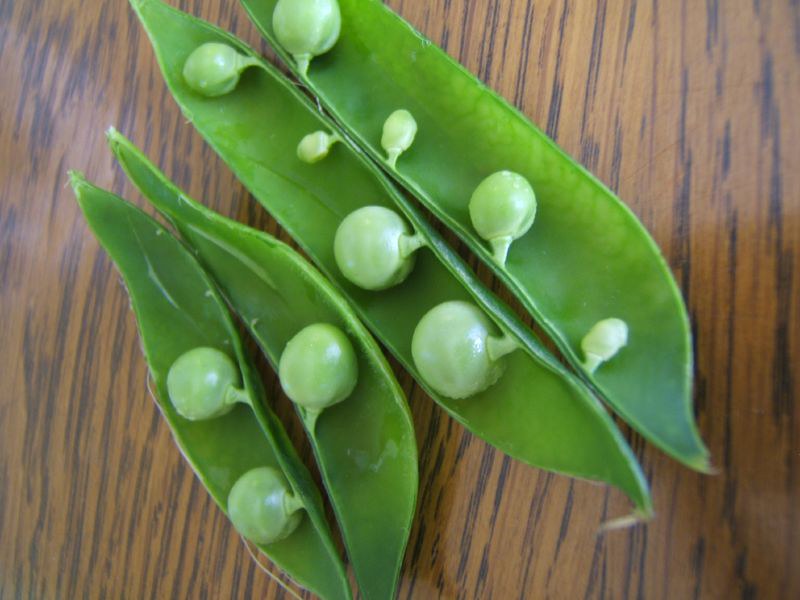In the image, we see two pea pods lying open on a medium brown laminate table with prominent black striations, giving it a richly textured appearance. The table's newness and sleek surface provide a stark contrast to the vibrant, glossy, Kelly green of the pea pods. Each pod appears unnaturally perfect, likely computer-generated, as evidenced by their flawless, smooth edges and vibrant color.

The pea pod on the left contains three peas: two on the left side and one on the right. A delicate stem is still attached to this light green pod. The pod on the right is larger and houses eight peas, symmetrically arranged with four on each side. Interestingly, the peas on both sides of this pod diminish in size towards the top and bottom, with the two central peas being the largest. The meticulous arrangement and the shiny, almost plastic-like appearance of the peas and pods further contribute to the impression that this is an idealized representation rather than real produce. There is no text in the image, allowing the striking visual details of the pea pods and table to fully capture the viewer's attention.